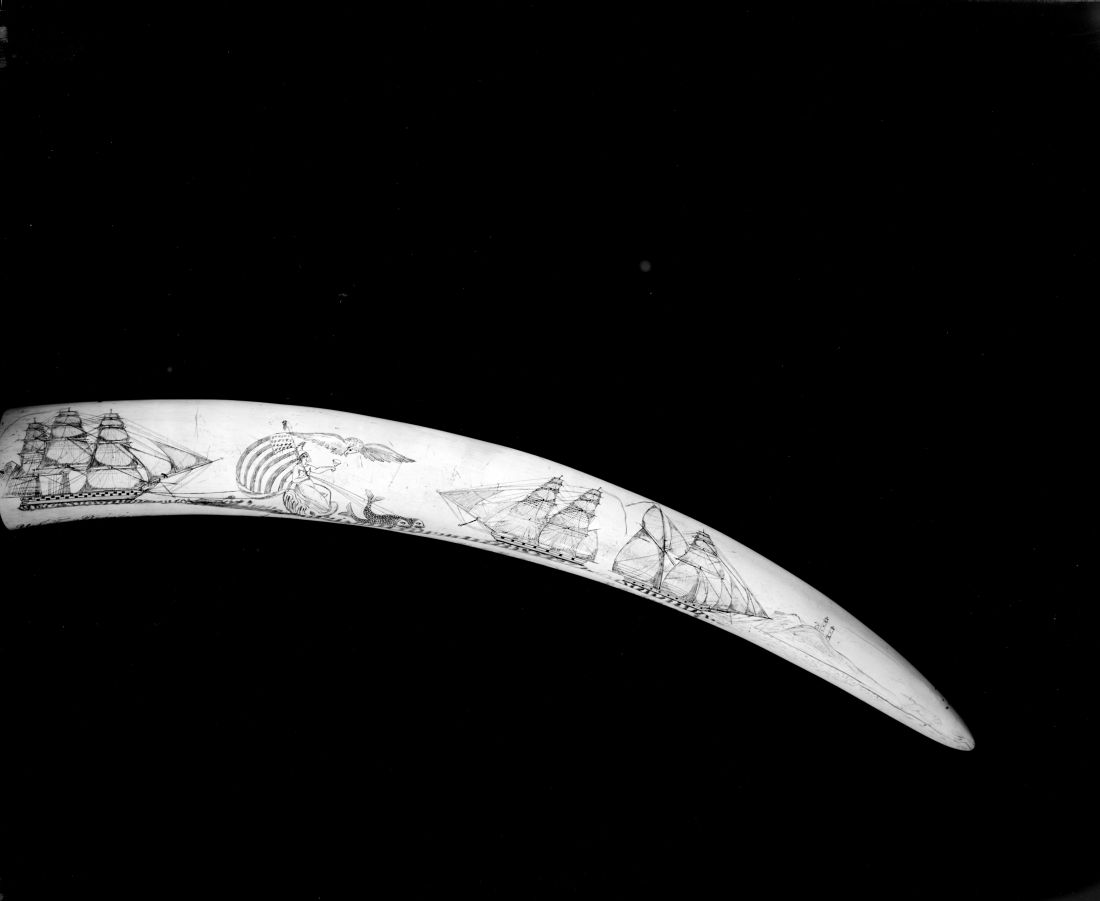The image features an antique piece of scrimshaw set against a solid black background. The primary focus of the image is an intricately etched, large walrus tooth ivory. The object, which dominates the center of the image, starts at the left middle edge and curves downward to the right, tapering to a rounded point. The scrimshaw's white surface is adorned with detailed etchings of multiple galleon ships, evident by their multiple sails and large structures, conveying a strong nautical theme. Positioned prominently on the flat end of the tusk is a finely detailed galleon ship. Adjacent to this, there is an intricately sketched scene featuring an 1800s period American woman, identifiable by her pointed hat and the American flag draped over her shoulder. She is depicted offering a cup to an eagle, while being pulled by stylized fish in the water. The other two galleon-like ships further enhance the maritime feel, emphasizing the historical and artistic value of this scrimshaw piece. The etchings, devoid of any text, utilize only shades of black, white, and gray, highlighting the artisanal craftsmanship and age of the object.